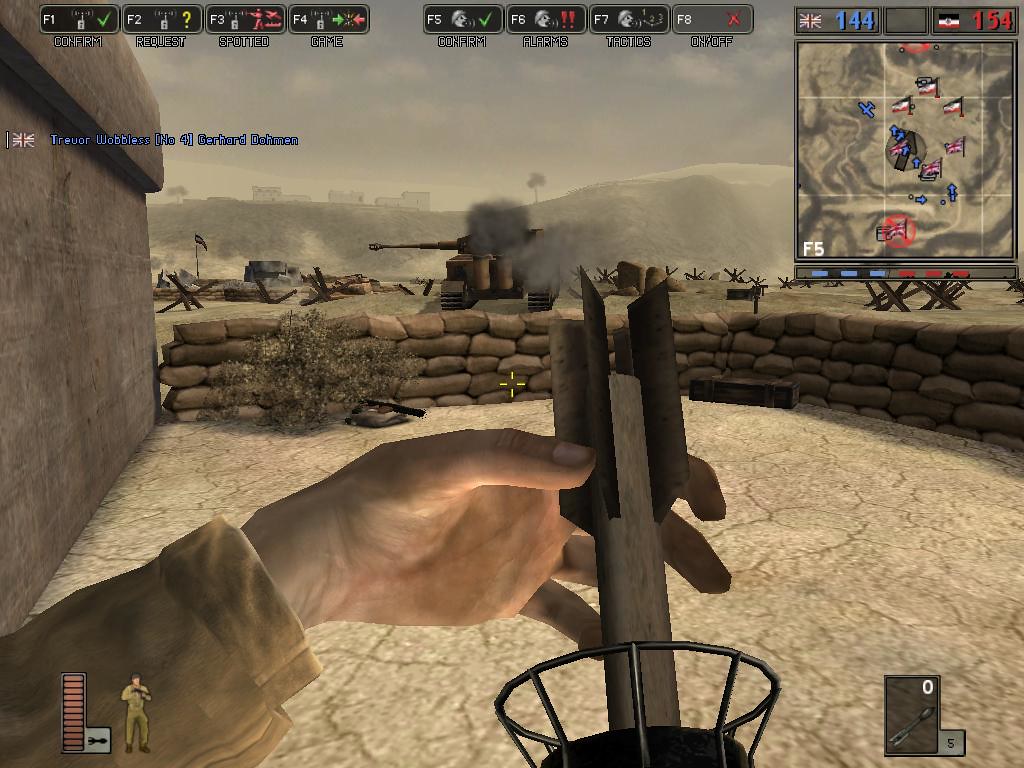The image is a 3D-rendered screen capture from a war game, showcasing a detailed heads-up display. In the center, the main character is seen loading a rocket into a missile-launching device, with a yellow crosshair positioned in the middle of the screen. The character, sporting a khaki long-sleeve shirt, uses his left hand to push the rocket into the launcher. A red, vertical health bar accompanied by a character paper doll is visible on the bottom left of the screen. The top right corner features a small map, displaying statistics for both teams involved in the game. The foreground reveals sandbags forming a barrier from the left to the right, while a concrete building stands on the left side. Directly ahead, above the crosshairs, is the rear view of a brown tank with smoke billowing from it, and its turret is turned to the left.